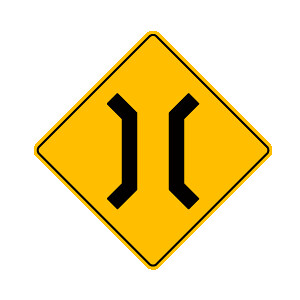This image depicts a small, yellow, diamond-shaped traffic sign with a thin black border set against a white background. The sign itself is positioned independently, not mounted on a pole. At the center of the sign is a black symbol, which consists of two thick black segments. Each segment starts from its respective upper corner and inclines towards the center, then goes straight down vertically before angling away from one another towards the bottom. The left segment begins at the upper left corner, while the right segment starts at the upper right. They form a mirrored arrangement resembling sectional couch backs facing each other or an entry path into something, likely indicating a bridge or a crossing.